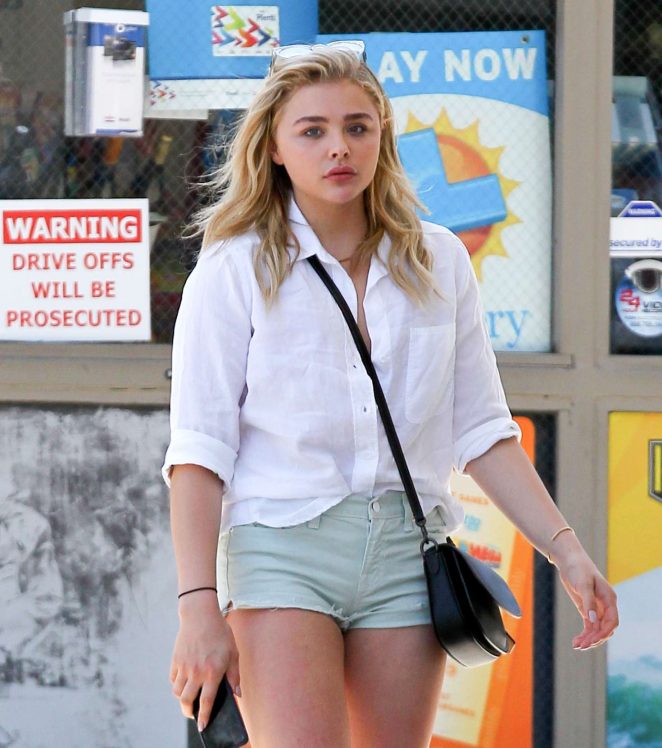The image depicts a young woman in her late teens, walking outside in front of a convenience store. She has fair skin and long blonde hair, contrasting with her dark eyebrows, dark eyes, and thick lips. She wears very short, mint green shorts and a white button-down shirt with rolled-up sleeves to her elbows, featuring a chest pocket. Her accessories include a small black purse draped across her right shoulder, hanging at her left thigh, a black rubber band around her right wrist, and a thin gold bracelet on her left wrist. She is holding a black mobile phone in one hand. Behind her, a fence with various signs is visible, including a white and red notice that reads, "Warning: Drive-Offs Will Be Prosecuted," and a white, blue, and yellow lottery sign that says "Play Now." The entire image is brightly lit by natural light, highlighting the vibrant colors and clear details of the scene.